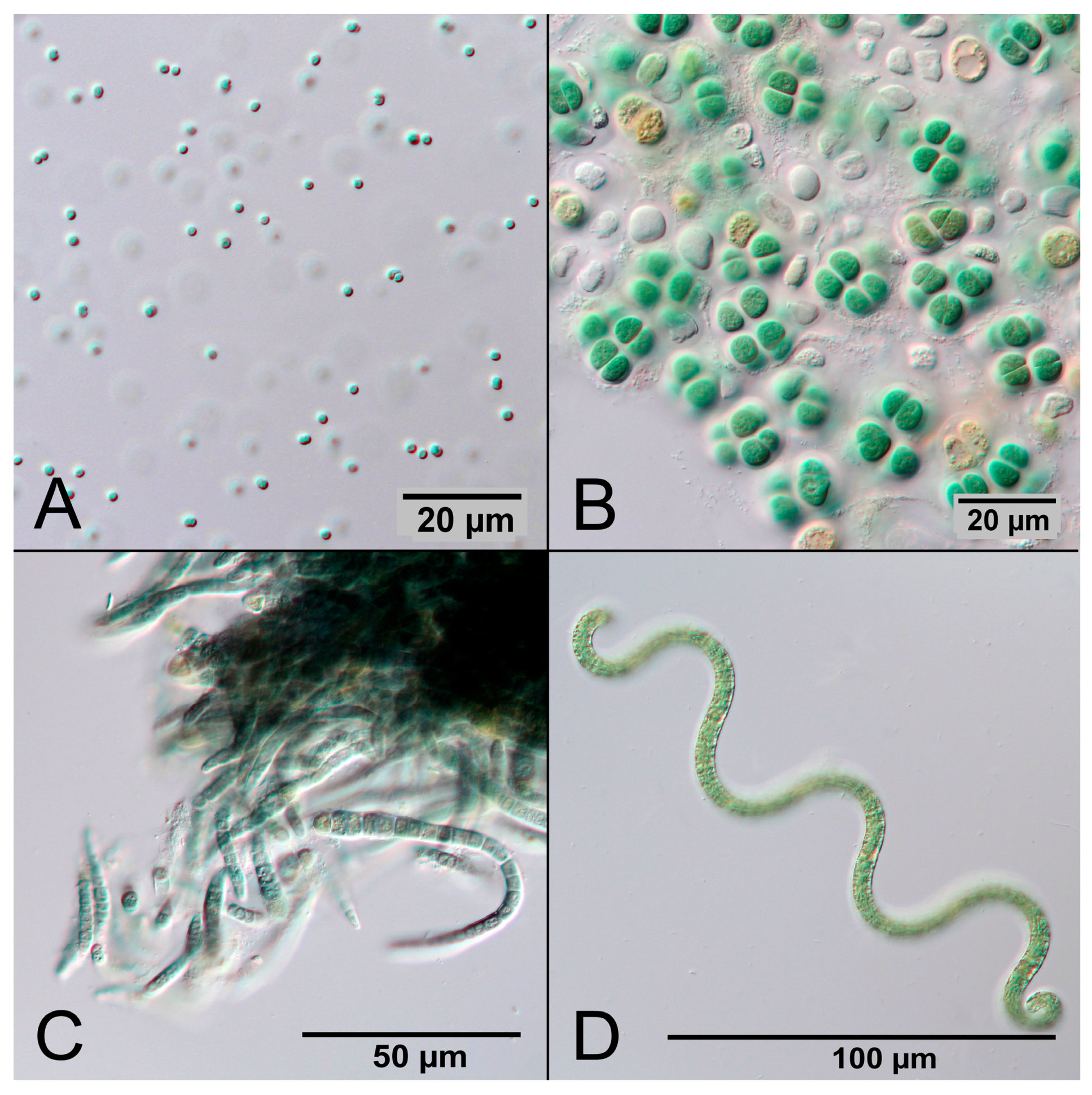This image is composed of four equal-sized squares, each labeled with a different letter and displaying microscopic details against a gray background. 

- The top left square, labeled "A" and marked with "20 µM", features small greenish dots scattered across a gray background. 

- The top right square, labeled "B" and also marked with "20 µM", contains larger green spots clustered together, along with some smaller yellow, tan, and white substances of varying shapes.

- The bottom left square, labeled "C" and marked with "50 µM", displays squiggly black, green, and white lines of various shapes and sizes against its gray background.

- The bottom right square, labeled "D" and marked with "100 µM", has a long, snake-like green object that appears thin, curly, and slightly blurry, surrounded by some white substance.

The overall feel suggests these are drawn from a microscopic view, potentially of bacteria, mold, or some other microorganisms, giving a detailed and varying depiction across the different squares.